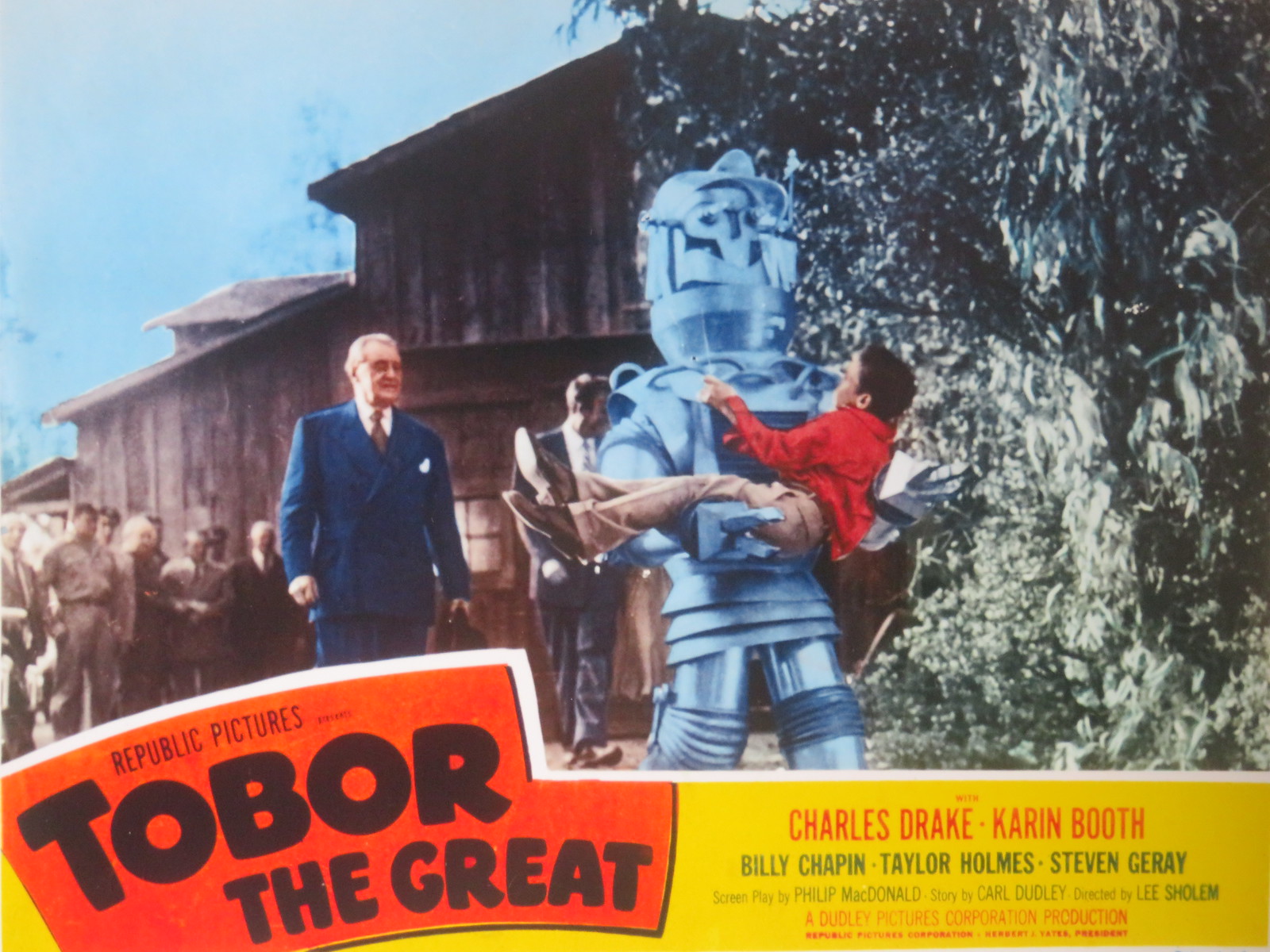The image is an old and somewhat peculiar movie poster from "Tobor the Great," presented by Republic Pictures Corporation. The main focus of the poster is a silver-colored robot, much larger than the other characters, holding a small boy who is dressed in slacks and a red shirt. Behind the robot, an older man in a blue suit, possibly a figure of authority, gazes at the boy. The background features a wooden house and a tree on the right side. At the bottom of the image, black text on a red backdrop lists the movie details: "Republic Pictures presents Tobor the Great," starring Charles Drake, Karen Booth, Billy Chapin, Taylor Holmes, and Stephen Gray. The smaller font at the bottom credits the screenplay by Philip Macdonald, story by Carl Dudley, and direction by Lee Sholem, noting it as a Dudley Pictures Corporation production.